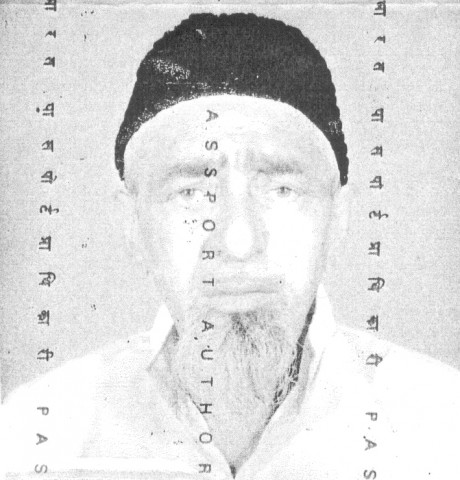The black and white photo features an older, pale-skinned white man, likely in his 40s or 50s, wearing a black knit beanie. His thick, bushy eyebrows frame a pair of empty, sad eyes. The man's expression is notably somber, with no hint of a smile—his mouth, adorned with quite large lips, is set in a neutral line. Facial hair is prominent, including a large goatee consisting of grayish hair hanging from his chin. He is dressed in a white polo shirt with a propped-up collar, exposing the top part of his chest due to the V-neck design. The image is very bright with minimal contrast, making details somewhat challenging to discern. Additionally, there is a watermark, along with three lines of symbols and vertical lettering, one of which references "passport authority." The background of the photo is grey, adding to the stark and slightly grim atmosphere of the shot, which resembles a passport or mug shot photo.